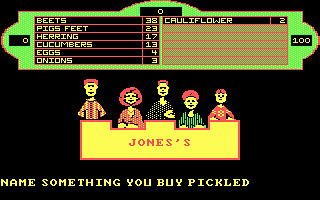This image is a screenshot from a vintage video game inspired by the popular television show, Family Feud. The game interface closely mimics the TV version, featuring a prominent scoreboard at the top where participants guess answers to survey questions. In this particular scene, the question posed to the players is "Name something you buy pickled," with answers including beets, pig's feet, herring, cucumbers, eggs, onions, and cauliflower. Displayed on the screen are two family teams: the Joneses, consisting of five members of varying ages – adults, younger individuals, and middle-aged participants. The current score shows zero points on the left side versus 100 points on the right side. This early screenshot of the game captures the nostalgic essence and graphical style of vintage video games, echoing the excitement and popularity of the original Family Feud TV show.